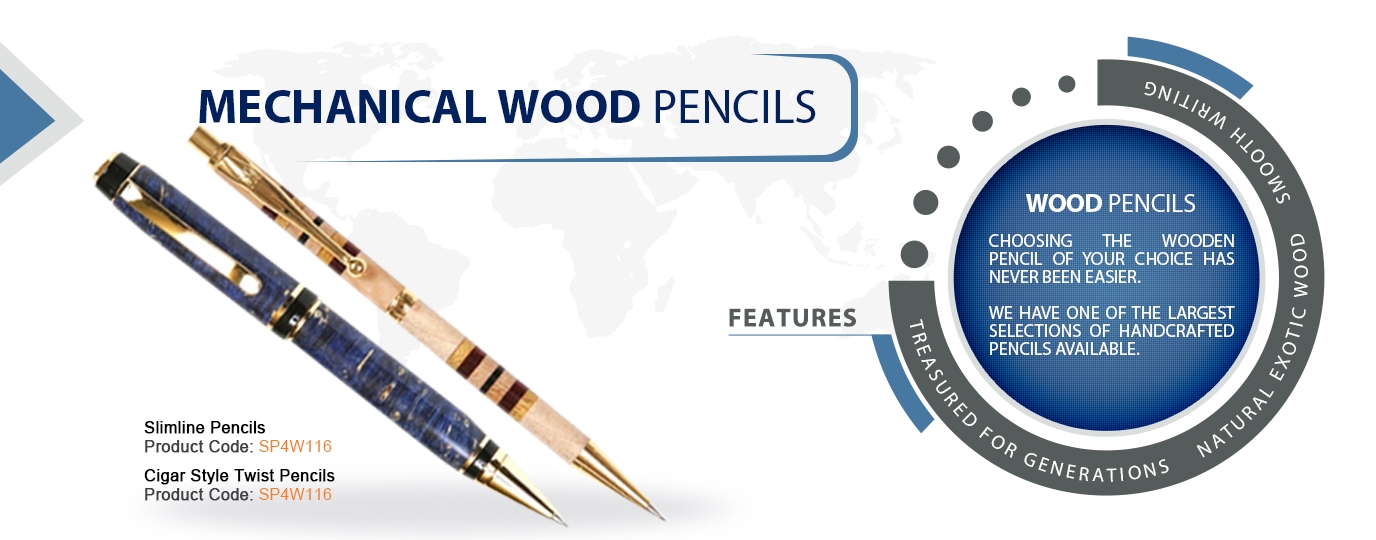This advertisement showcases two distinct mechanical wood pencils displayed diagonally from left to right. The first pencil, characterized as a Slimline Pencil with product code SP4W116, features a sleek design crafted from light brown wood with darker brown stripes. The second, wider pencil is a Cigar Style Twist Pencil, also with product code SP4W116, and is made from blue wood adorned with gold trim. On the right side of the advertisement is a circular emblem adorned with dotted accents around its outline. The outer rim of the circle reads "Treasured for Generations," "Natural Exotic Wood," and "Smooth Writing." Inside the circle, against a blue background with white text, it announces "Wood Pencils," proclaiming that "Choosing the wooden pencil of your choice has never been easier." The advertisement further emphasizes that they offer "one of the largest selections of handcrafted pencils available."